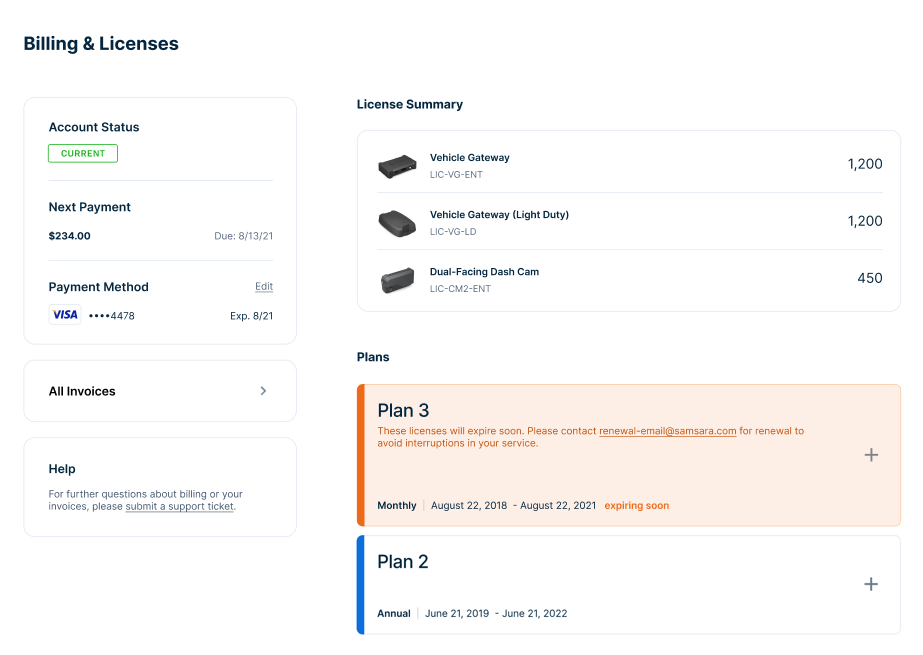This is a highly detailed depiction of a checkout page on a website featuring three main sections on a white background. 

In the top left corner, black text reads "Billing & Licenses." Below this headline, there are three distinct sections each outlined with a thin gray border and rounded corners.

### First Section: Account Status
At the top left of this section, "Account Status" is written in black text. Below this, there's a button with a white background, a green outline, and green text that says "Current." Underneath this button, a thin gray horizontal line separates the subsequent details.

Next, "Next Payment" is listed in black text, followed by the amount of "$234" on the left side of the line. To the right of this amount, light gray text notes "Due: $813.21." Another thin light gray line runs beneath these details.

Further down, "Payment Method" is displayed in black text in the top left. Below this, a Visa logo appears on a white background. Positioned next to the logo are four gray dots indicating hidden card numbers, followed by the last four digits "4478." In the bottom right corner of this section, "Exp. 08/21" is noted. The word "Exp." is abbreviated and followed by a period. Below this, light gray text reads "Edit," which is underlined, indicating it is a clickable link.

### Second Section: All Invoices
After a small area of negative space, the next section features a light gray outline. "All Invoices" is centered left in black text, and a dark gray arrow pointing right is displayed on the far right.

### Third Section: Help
The final section is labeled "Help" in dark gray text at the top left corner. Beneath this, a two-line paragraph in light gray text states, "For further questions about billing or your invoices, please submit a support ticket." The phrase "Submit a support ticket" is underlined to signify it is a clickable link.

### License Summary
To the right side of the page, "License Summary" is written in black text at the top left. Beneath this heading, a panel with a thin light gray outline and rounded corners is present. This panel contains three rows, each featuring a picture of the product on the left, the product title to the right of the image, a single line of light gray text beneath the title, and the price displayed on the far right.